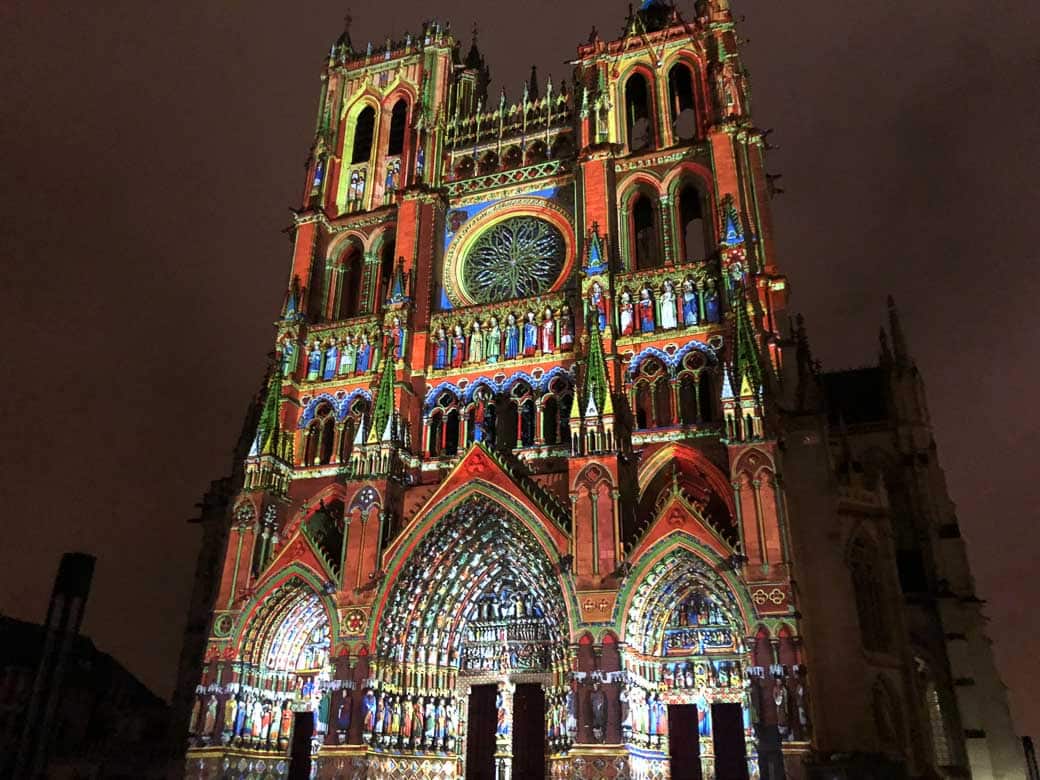The photograph depicts the iconic facade of a cathedral, possibly Notre Dame Cathedral, renowned for its recognizable Gothic architecture. The scene is captured at twilight, with the sky bathed in a brown hue, while the bottom part of the structure is illuminated vibrantly, casting a dramatic juxtaposition against the darkened surrounding buildings.

The facade, detailed with intricate and ornate carvings, showcases rows of statues, each adorned in various colored robes—blue, red, yellow, and green, adding to the building's vibrant appeal. Central to its design are the three Gothic arch doorways, with the middle arch standing the tallest and widest. Above the doors, a round stained glass window, commonly known as a rose window, is prominently featured along with additional stained glass panels that decorate the façade and arches. 

Crucifixes are mounted on the walls and ceilings, enhancing the religious significance of the edifice. The cathedral’s structure and ornate details, including the colorful artistry of the stained glass and carved figures, reflect an awe-inspiring level of craftsmanship, solidifying its status as a monumental and iconic piece of architecture.